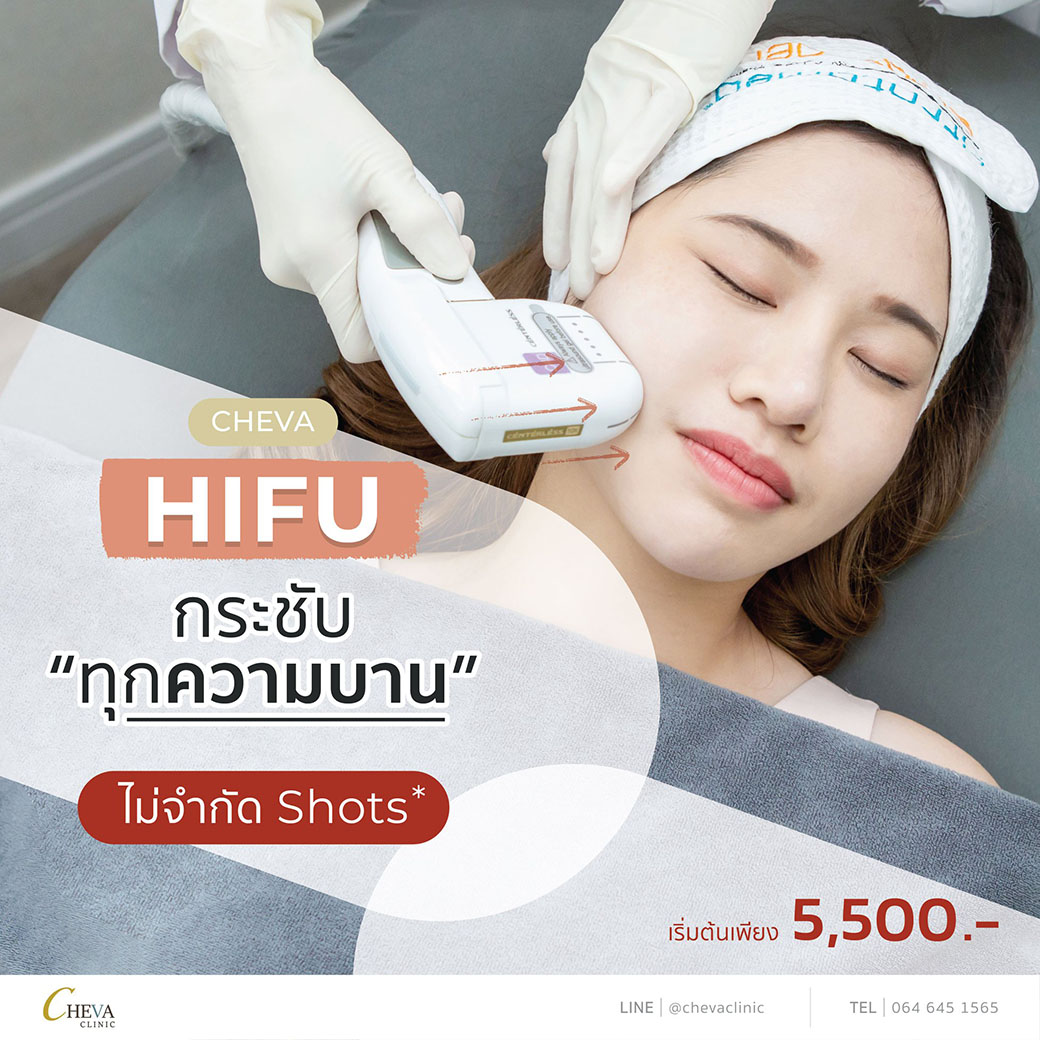The image is a detailed advertisement for CHEVA, a clinic or spa. The ad features a young woman, likely of Asian descent, with closed eyes and a serene expression, lying on a treatment table with a blue towel draped over her body and a white headband keeping her brown hair away from her face. A clinician wearing white latex gloves is administering a laser device or similar treatment to her cheek, indicated by light red arrows pointing from the device to her face. The setting appears to be a professional clinic, suggesting the procedure is aimed at enhancing skin appearance, possibly through exfoliation or red light therapy. The advertisement, which spans 9 inches by 9 inches, includes text in a non-English language with a price and the procedure's name that are not decipherable. Key details include the prominent CHEVA branding, social media links, and a contact number in the lower right corner: 064-645-1565.